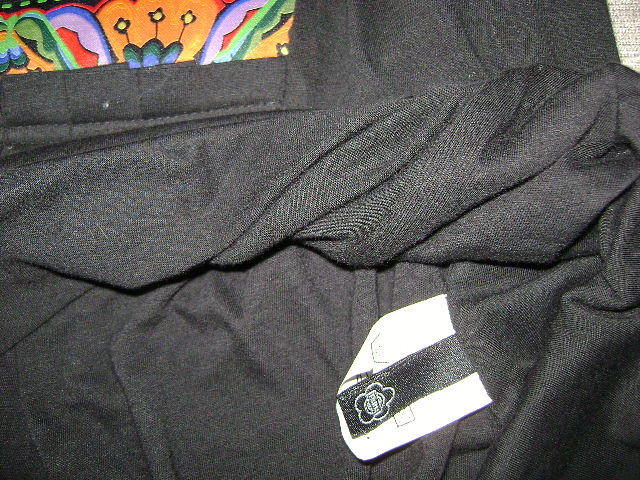The image depicts a black piece of fabric, intricately woven with visible large threads and pleats at the bottom, suggesting a quilt-like construction. On the right-hand side, a tag with white and black hues features a distinct asterisk-like floral outline and white writing in its black strip. The top left-hand corner of the image is vibrant with colors—orange, purple, green, blue, yellow, and red—forming a background decorated with stars and three small flowers. These flowers have black petals and yellow centers, nestled amidst a colorful and lively backdrop.